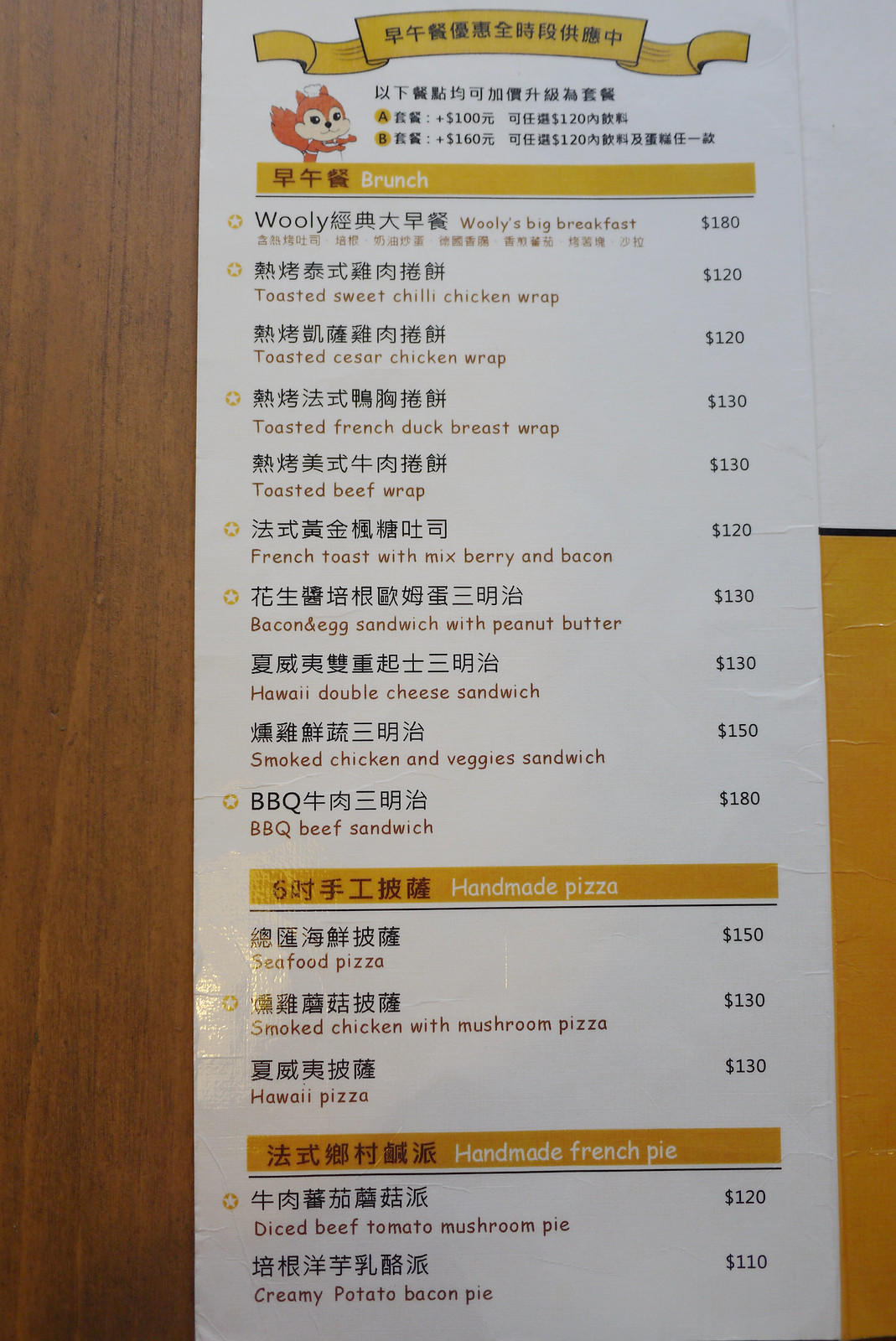The image displays a tall menu with a golden banner at the top featuring text in either Chinese or Japanese. On the left side of the banner, there's a red 'Chinmung' logo. The menu lists various food items along with their respective prices:

- Woolly’s Big Breakfast: $180
- Toasted Sweet Chili Chicken Wrap: $120
- Toasted Caesar Chicken Wrap: $120
- Toasted French Duck Breast Wrap: under $30
- Toasted Beef Wrap: under $30
- French Toast with Mixed Berries and Bacon: $120
- Bacon and Egg Sandwich with Peanut Butter: under $30
- Hawaiian Double-Cheese Sandwich: under $30
- Smoked Chicken and Veggie Sandwich: under $50
- BBQ Beef Sandwich: under $80
- Seafood Pizza: under $50
- Smoked Chicken with Mushroom Pizza: under $30
- Hawaiian Pizza: $130
- Diced Beef Tomato Mushroom Pie: under $20
- Creamy Potato Bacon Pie: under $10

Each category is clearly listed, providing a comprehensive view of the available menu options and their prices.